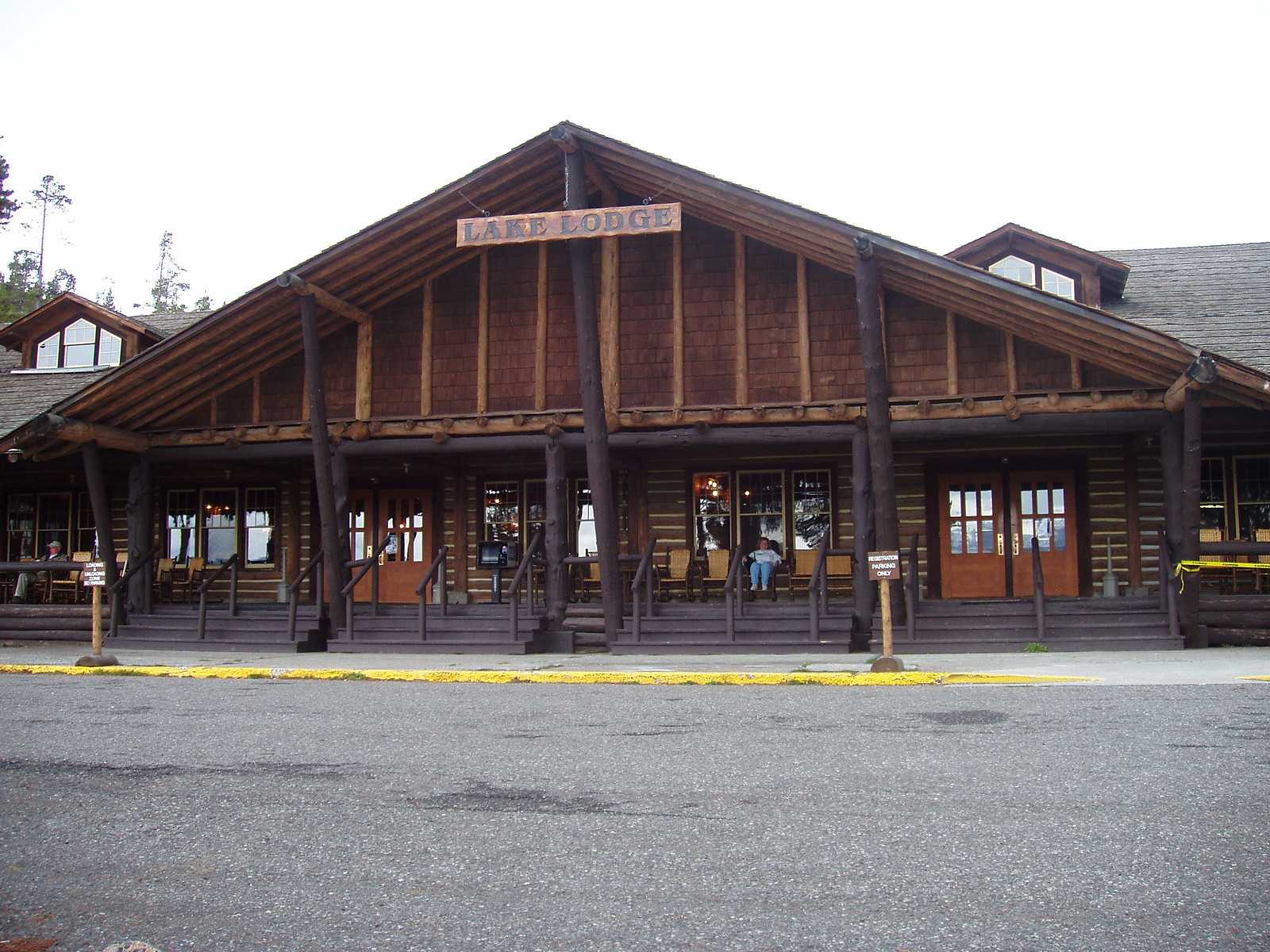The image captures a traditional wooden lodge named "Lake Lodge," identified by a prominent sign in serif font hanging above. The lodge, constructed primarily of dark wood with large, log beams, exudes a classic cabin aesthetic. The building's exterior features architectural elements such as gables with small roofs on both the left and right sides. The lodge has multiple entry points, including a set of two wooden doors and three staircases, highlighting its spacious frontage.

In front of the lodge runs a sidewalk bordered by a yellow-painted curb, indicating no parking. Two posted signs and a newspaper dispenser are also visible along the street. Several wooden chairs or benches line the front porch, occupied by at least two individuals— a man on the left and a woman on the right— who seem to be enjoying their time outside. The sky overhead suggests a bright yet overcast day, as it appears mostly white without distinct colors.